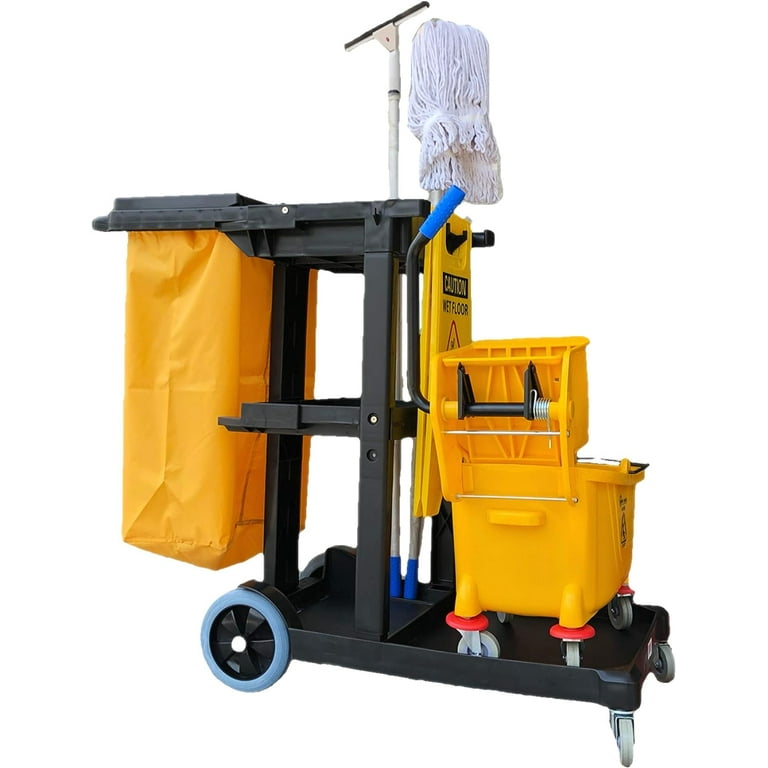The image features a janitorial cleaning cart set against a featureless white background, reminiscent of catalog illustrations. The cart, seemingly constructed from steel, is equipped with two large, fixed blue-tired wheels at the back and two smaller, pivoting casters at the front for easy maneuverability. Loaded onto the cart, from left to right, are a large yellow trash bag holder for waste collection, a black plastic frame that houses cleaning tools including a long-handled window squeegee and a mop with white strands, and a folded caution "Wet Floor" sign. At the forefront of the cart is a yellow mop bucket with an integrated wringer. The entire setup appears brand new, indicating it could be an advertisement for a supply website.